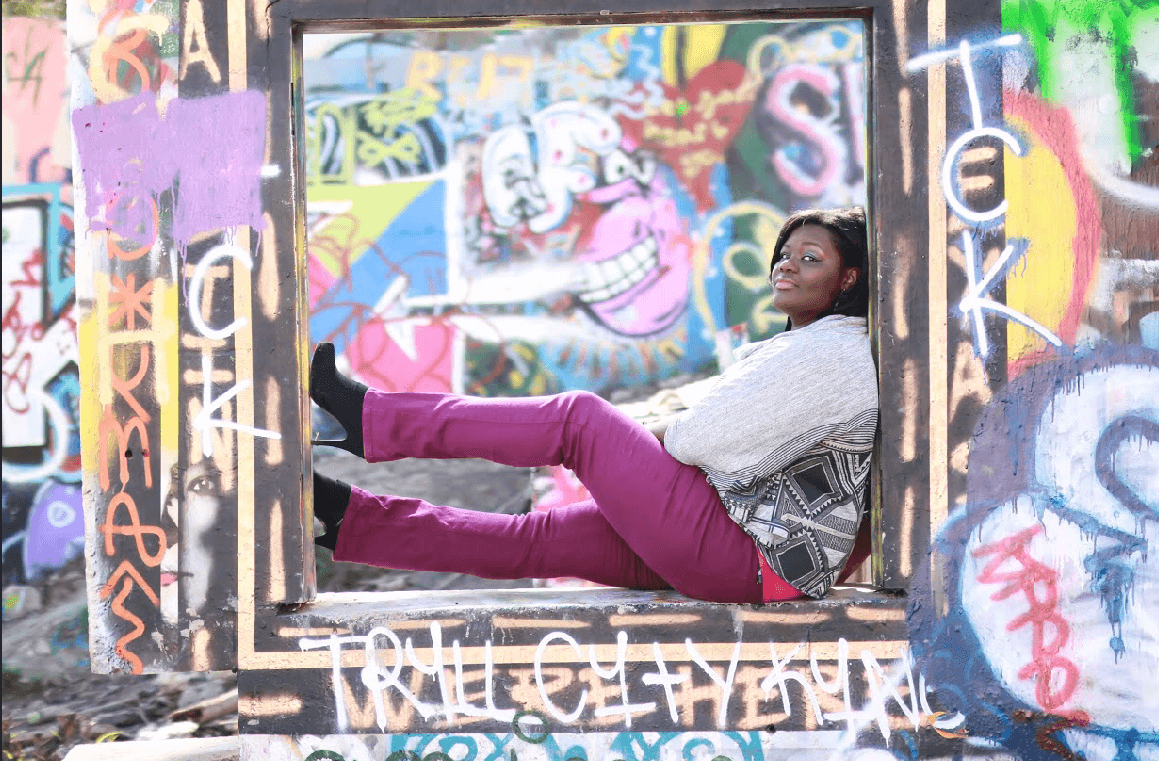A young African-American woman with short, shoulder-length black hair and side-swept bangs sits stylishly in an open rectangular hole in a concrete wall, surrounded by a heavily graffitied, roofless structure. She sports blue eyeshadow, high-heeled black shoes, and vibrant purple jeans. Her grey sweatshirt, adorned with tribal or geometric designs in white and black, matches the edgy and creative backdrop of the image. With her feet up against one side of the opening and her back braced against the other, she gazes directly at the camera with a calm and composed expression. The wall she sits in, and the one behind her, are both covered in layers of graffiti, including a prominent large face, possibly purple, and an assortment of indistinct words in various fonts. The scene is chaotic yet intriguing, with miscellaneous graffiti art adding a raw urban charm to the composition.